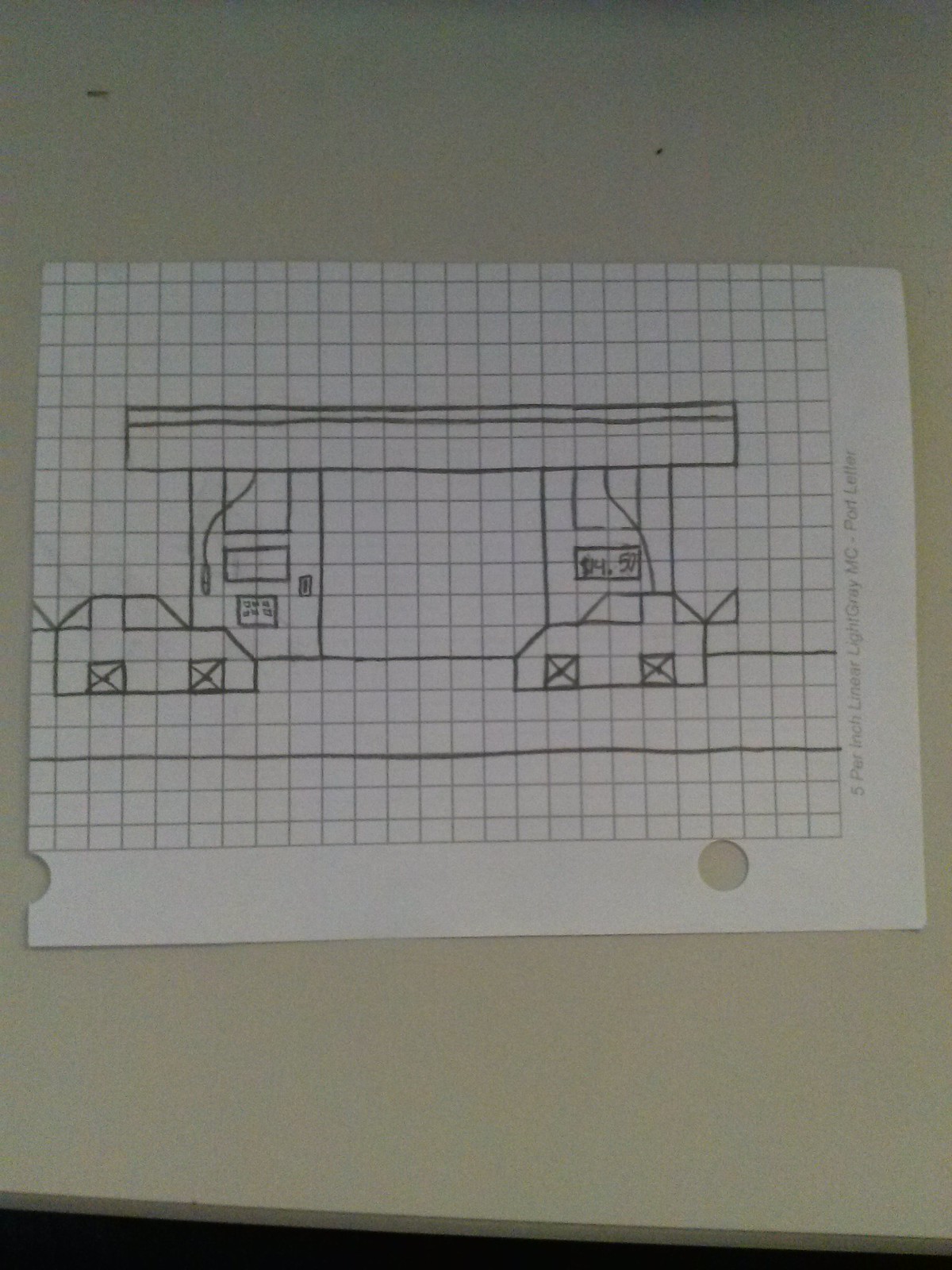This image depicts a detailed hand-drawn pencil illustration on a white sheet of graphing paper, which is placed on a white, smooth-surfaced table. The paper, characterized by its grid pattern often used in math and architecture, has hole punches on the side, indicating it might have been part of a notebook. The drawing features two boxy cars positioned in front of gas pumps under an awning, with one car actively filling up at $4.50 per gallon indicated on the pump, and the other car in the process of pulling up. The cars sport square tires marked with X's in the centers, and the meticulous alignment of shapes with the grid lines showcases the artist's careful attention to detail. The scene is illuminated against the darkness that shrouds the floor beyond the table's edge, bringing focus to the simplicity and precision of the artist's work.